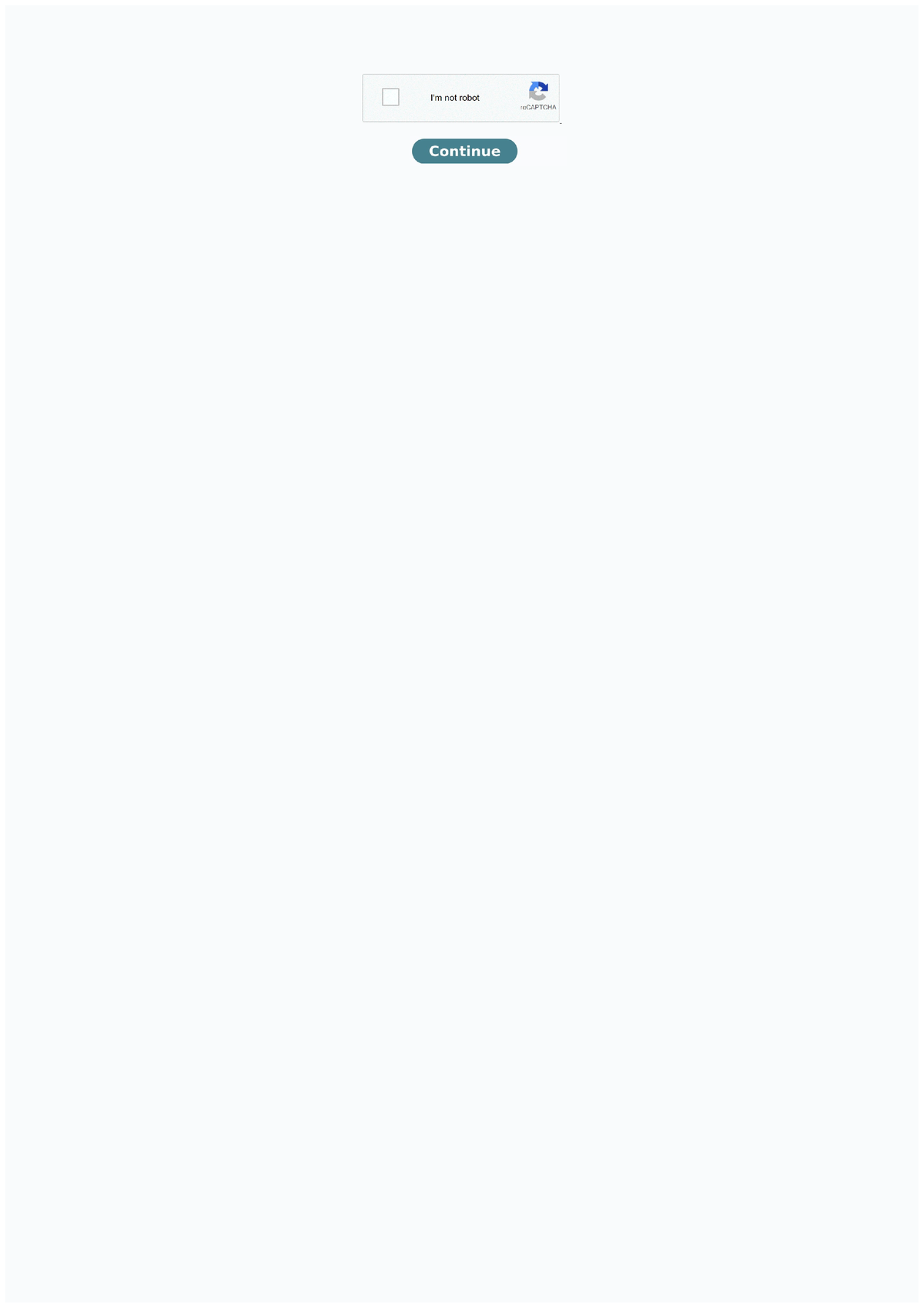Screenshot depicting a minimalist web page with an entirely white background. At the very top center, occupying about 10% of the screen, is a CAPTCHA verification prompt. Central to this prompt is a white rectangle outlined in black. Inside this rectangle, on its left side, is a smaller white square similarly outlined in black. Centered within the rectangle, black text reads: "I'm not a robot." On the right side of this rectangle is the reCAPTCHA logo, depicted as a circle composed of three arrows arranged clockwise. The bottom arrow is gray and points upward, connecting to a light blue arrow pointing to the right, which then leads to a dark blue arrow pointing downward. Below the logo, light gray text reads: "reCAPTCHA." Directly beneath this rectangle lies an oval button in a tealish blue hue, featuring the word "Continue" in white lettering.